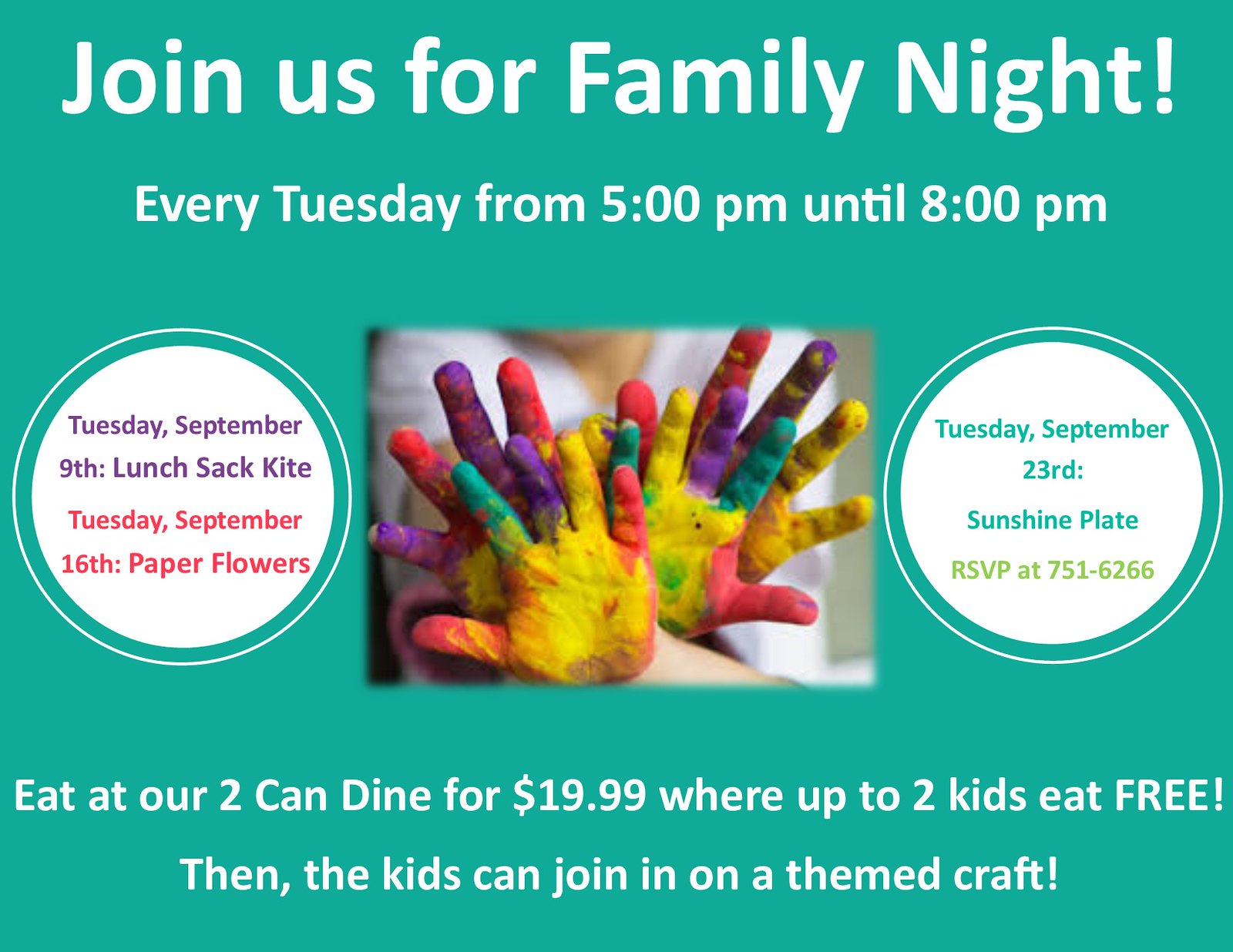The advertisement poster features a sage green background with the bold white heading "Join us for Family Night!" at the top. Directly beneath this, in smaller white print, it announces, "Every Tuesday from 5 p.m. until 8 p.m."

The center of the poster contains an eye-catching image depicting several hands painted in a variety of vibrant colors including yellows, aquas, purples, blues, and pinks. The hands are held up together as if giving jazz hands.

On the left side of the image, there is a white-outlined circle filled in white, listing upcoming craft activities in purple text. It reads: 
- "Tuesday, September 9th - Lunch Sack Kite"
- "Tuesday, September 16th - Paper Flowers"

To the right of the painted hands, another circle displays:
- "Tuesday, September 23rd - Sunshine Plate"
- "RSVP at 751-6266" in shades of turquoise and green.

At the bottom of the poster, in white print, it advertises a special meal deal: "Eat at our 'Two Can Dine for $19.99' or up to two kids eat free! Then, the kids can join in on the themed craft!"